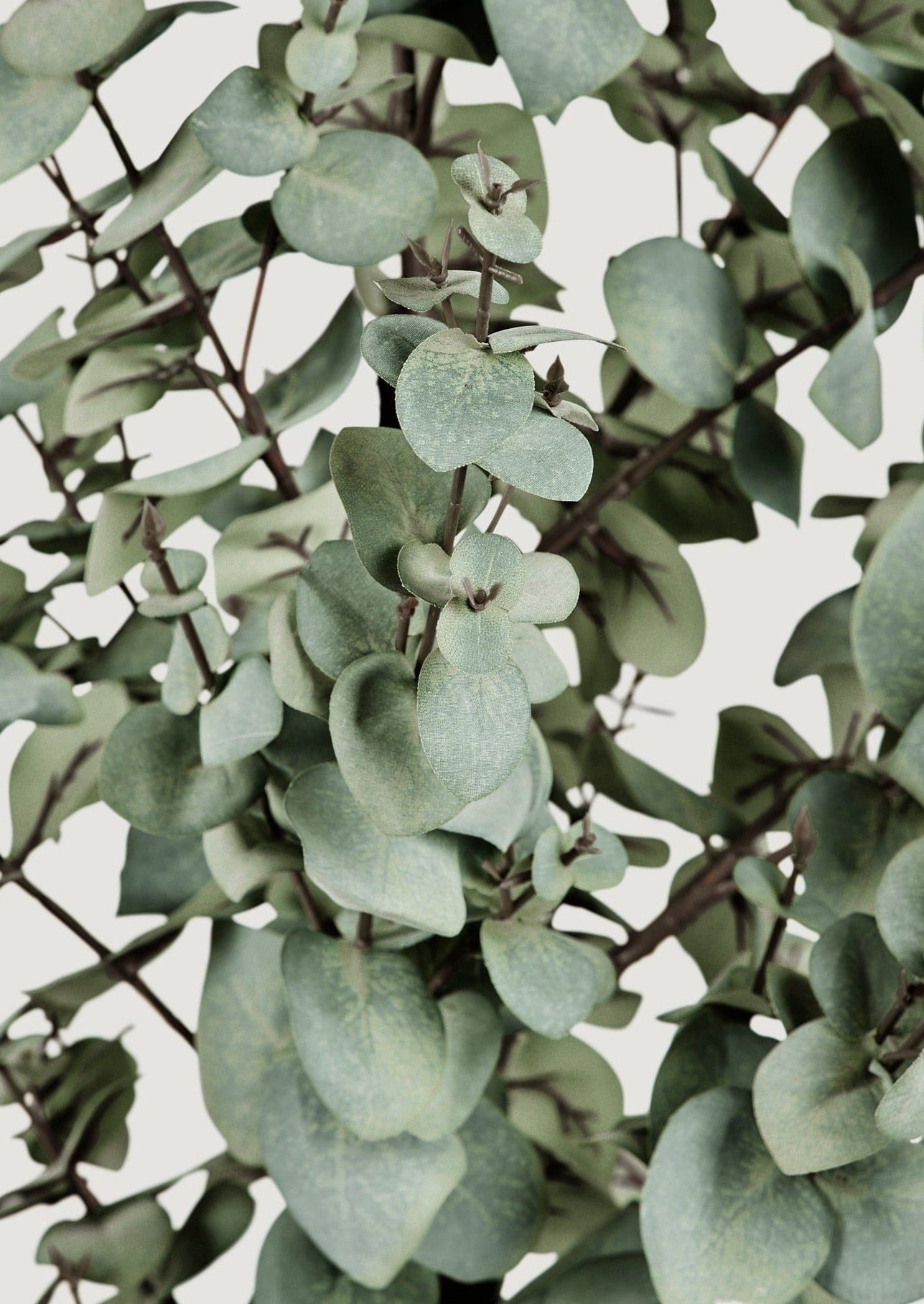The photograph is a tall, vertical image focusing on a single plant against a light gray background, which occupies the majority of the image. The plant appears to be a bush or small tree with thin, dark brown stems that are mostly straight, curving slightly outward. The branches are adorned with a multitude of green leaves of varying shapes and sizes, some exhibiting a speckled yellow hue and appearing slightly dirty, indicating a dry condition. The leaves have smooth edges, and there are no thorns. The background looks a bit foggy or edited, giving it a somewhat artificial appearance, suggestive of possible post-processing or Photoshop work to remove unwanted details. The primary subject, the plant, stands out prominently against the simple, monochromatic background, emphasizing its intricate details.